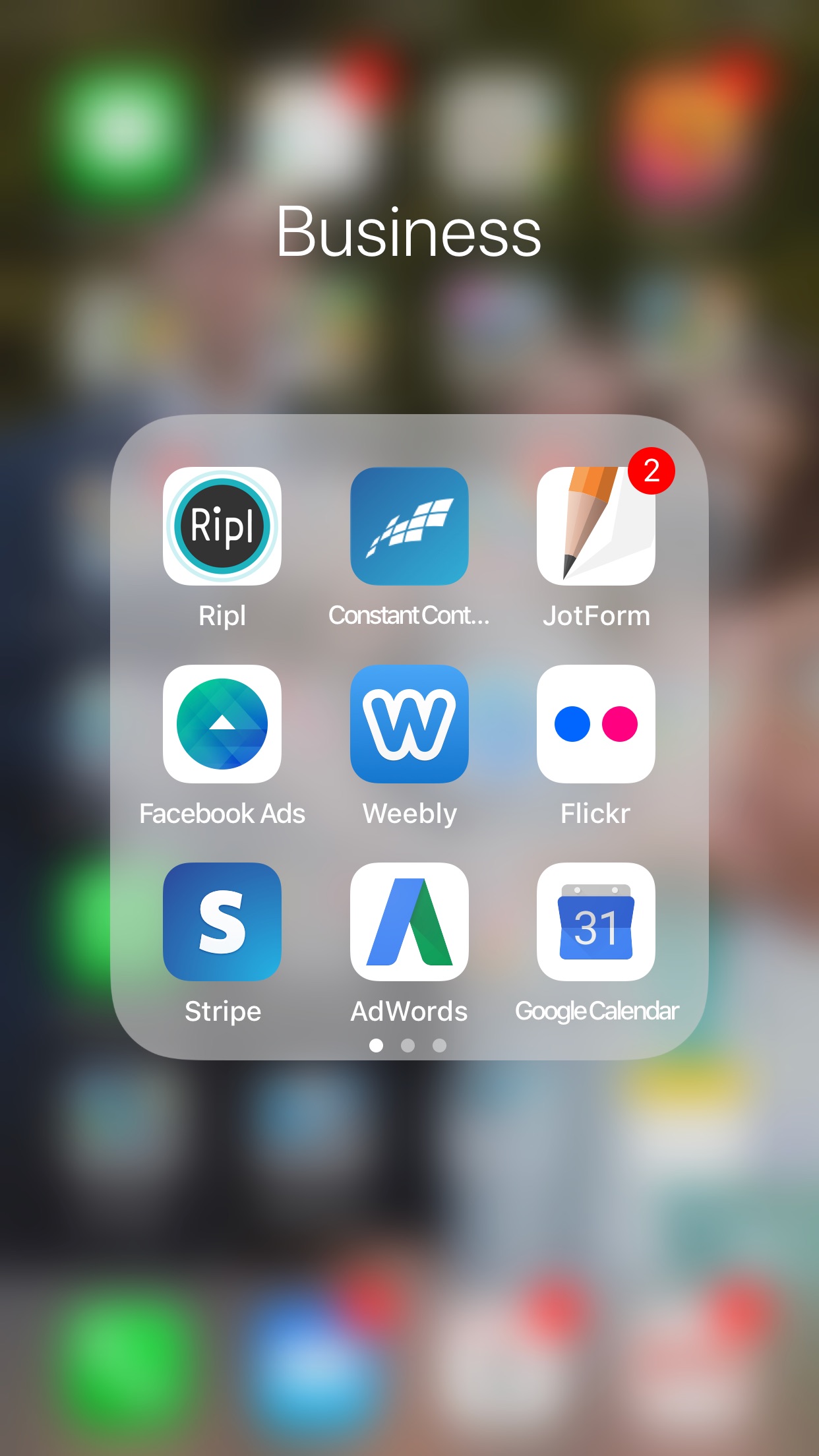A mobile device screen is displayed with a folder titled "Business" in white lettering at the top. The background of the screen appears to be soft-focused and slightly fuzzy. In the foreground, various business-related apps are organized within the folder. From left to right, the top row includes the following apps: Ripple (R-I-P-L), Constant Contact, and JotForm. The middle row features Facebook Ads on the left, Weebly in the center, and Flickr on the right. The bottom row displays Stripe at the far left, AdWords in the middle, and Google Calendar (with the number 31) on the right. Notably, the JotForm app shows a red notification badge with the number two, indicating two pending notifications. This collection of apps suggests a focus on business and productivity, conveniently grouped together for easy access on the user's phone.